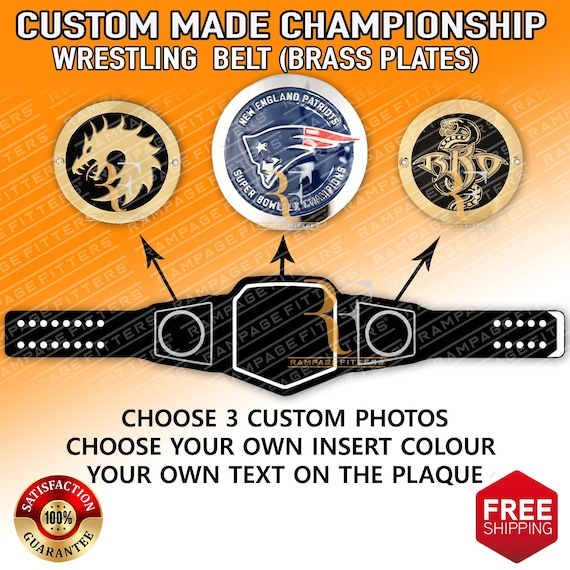This image is an advertisement for Rampage Fitters, promoting their custom-made championship wrestling belts with brass plates. At the top of the ad, "Custom-Made Championship Wrestling Belt (Brass Plates)" is prominently displayed in white on an orange background. Featured prominently in the center is a black leather wrestling belt with visible belt holes for fastening. The belt is designed to hold three custom brass plates, which are showcased below the text.

The centerpiece of the belt is a larger disc featuring a patriotic design with a blue background and a white border, emblazoned with "New England Patriots." On the left side of the belt is a smaller black circle edged in gold, depicting a majestic gold dragon facing left. The right side of the belt features another gold-edged black disc with intricate lettering, though the specific characters are difficult to discern.

The ad highlights that customers can "Choose three custom photos, choose your own insert color, your own text on the plaque." Additionally, it emphasizes a satisfaction guarantee with two red and gold insignias: one on the left declaring "Satisfaction 100% Guaranteed" and another on the bottom right indicating "Free Shipping."

Overall, the belt offers a striking combination of customizable features, allowing buyers to personalize their championship wrestling belts to their liking.